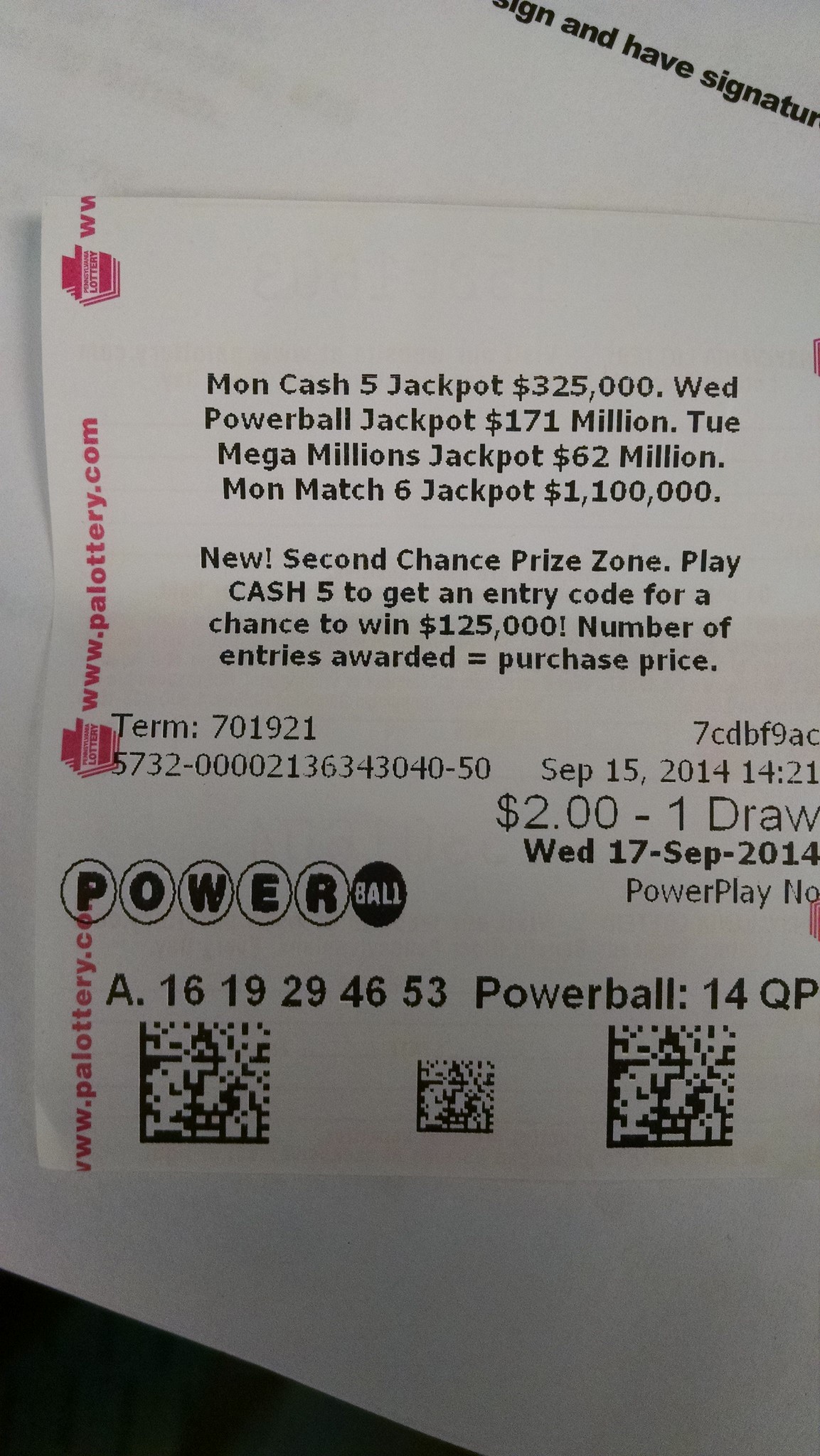The image features a detailed receipt for a lottery ticket, placed on a plain white surface. This ticket includes several lottery jackpot announcements: Monday's Cash 5 Jackpot at $325,000,000, Wednesday's Powerball Jackpot at $171,000,000, Tuesday's Mega Millions Jackpot at $62,000,000, and Monday's Match 6 Jackpot at $1,100,000,000. In bold, it also highlights a new Second Chance Prize Zone where playing Cash 5 grants an entry code for a chance to win $125,000, with the number of entries corresponding to the purchase price.

The ticket contains various identification and transaction details: Terminal number 701921, and a long unique identifier 5732-00002136343040-50. It indicates the purchase was made on September 15, 2014, at 14:21, priced at $2 for a single draw scheduled for Wednesday, September 17, 2014. The chosen numbers are 16, 19, 29, 46, and 53, with a Powerball number of 14QP. The top right corner features the web address "www.palottery.com" repeated three times vertically. The ticket also displays three QR codes at the bottom. The whole ticket is in black text on white paper, and in the background, a hint of the word "signature" appears in the upper right corner, with a grey corner suggesting the surface it sits on.